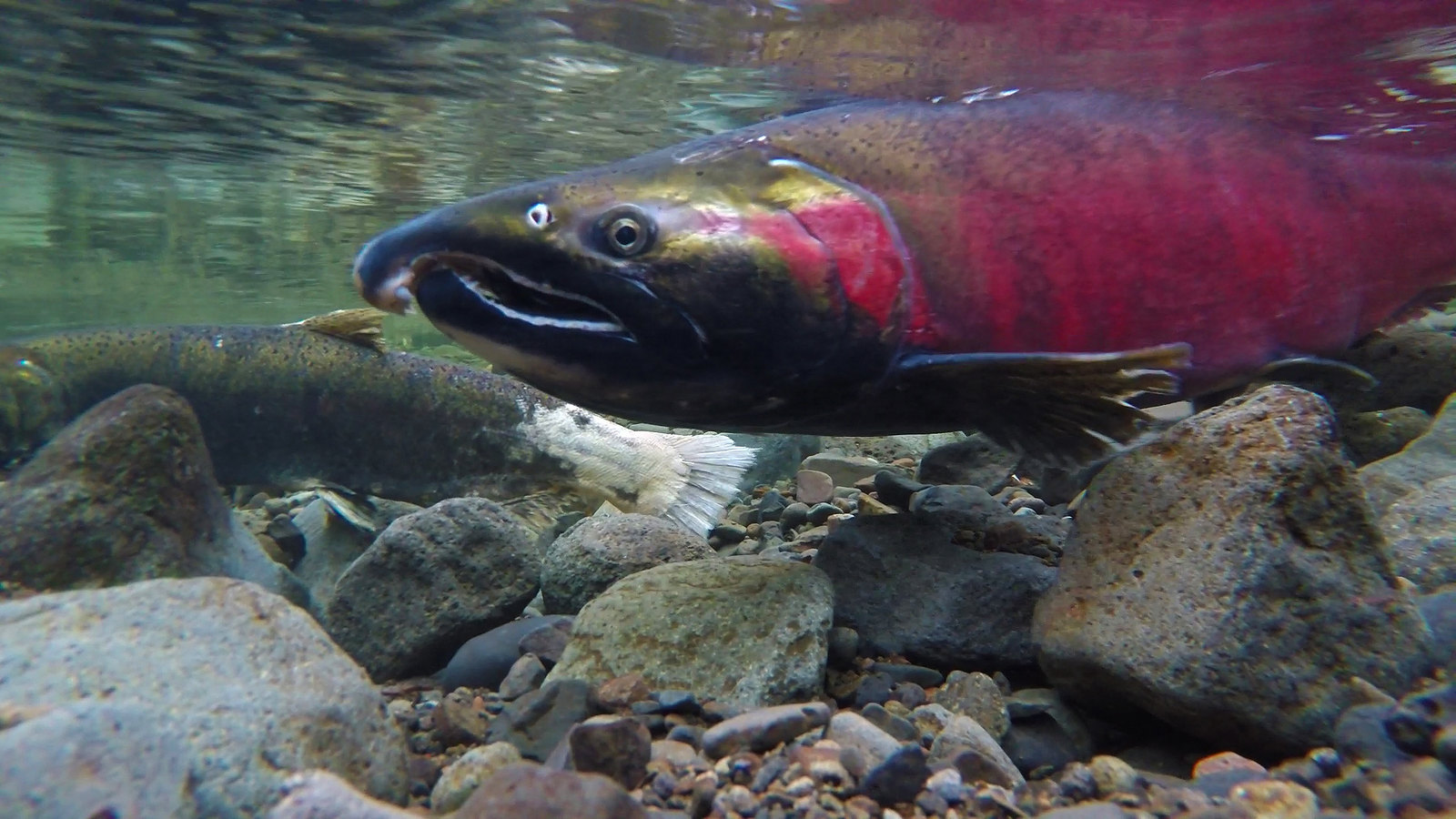This close-up underwater image captures two fish swimming in a shallow lake, characterized by its rocky bed, scattered with large and small rocks. The foreground features a prominent fish, with a hooked nose and an open mouth, swimming close to the lakebed. This fish is striking in its bronze hue with a greenish tint, adorned with vivid red markings stretching down its gills and sides, giving the impression of blood under the filtered light. Its fins brush against the rocks as it glides. To the left and in the background, another fish can be seen, whose body transitions from a greenish-bronze color to a white tail, though its face is not visible in the image. The surface of the water is noticeable, indicating the shallowness of the lake.